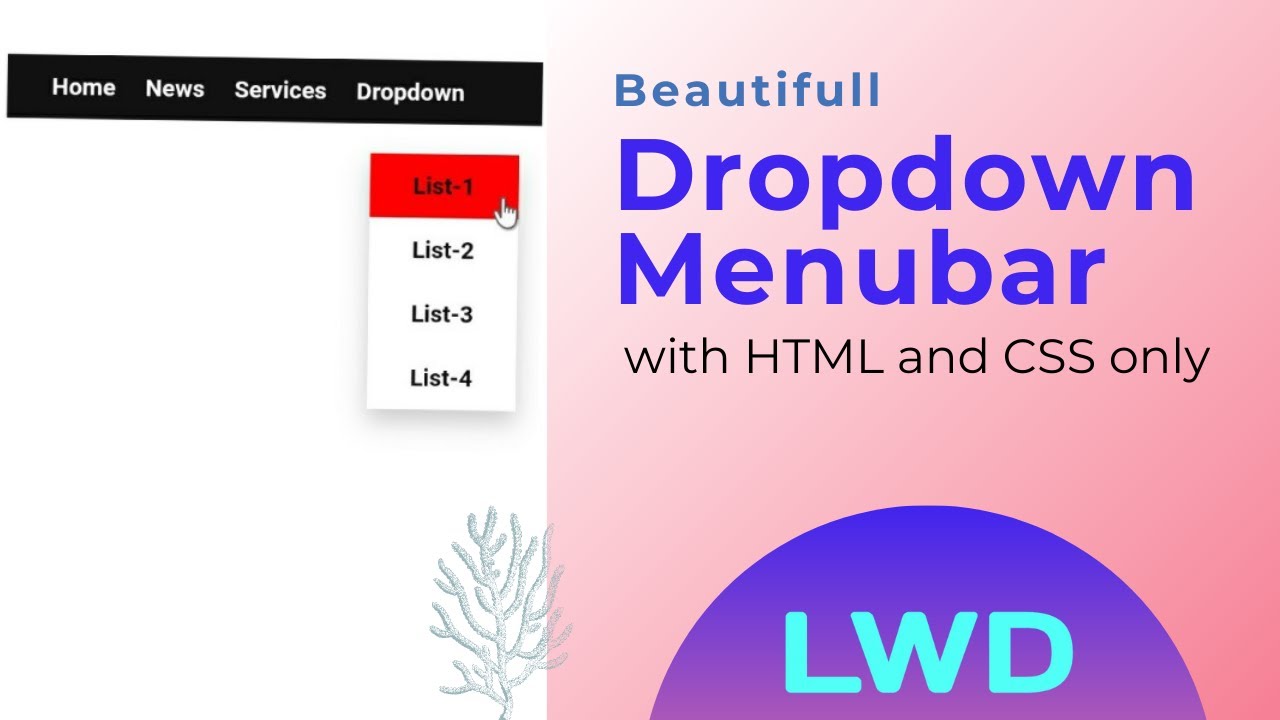The image depicts a webpage layout, showcasing four main navigation tabs labeled "Home," "News," "Services," and "Dropdown." When the "Dropdown" tab is expanded, it reveals a vertical list of four items: "List One," "List Two," "List Three," and "List Four." Beneath this dropdown menu is a concise white space area containing distinct visual elements. At the bottom, there's a slightly bluish image of a simple eye coral, adding a touch of marine aesthetics. To the left of the coral image, a pink square prominently features the word "Beautiful," misspelled with an extra "L" (light blue text). Below this, in large, separate lines of bold blue text, it reads "Dropdown Menu Bar," emphasizing a hierarchical structure. Completing the layout, a smaller text underneath mentions "with HTML and CSS only," indicating the technologies used to create the dropdown functionality.